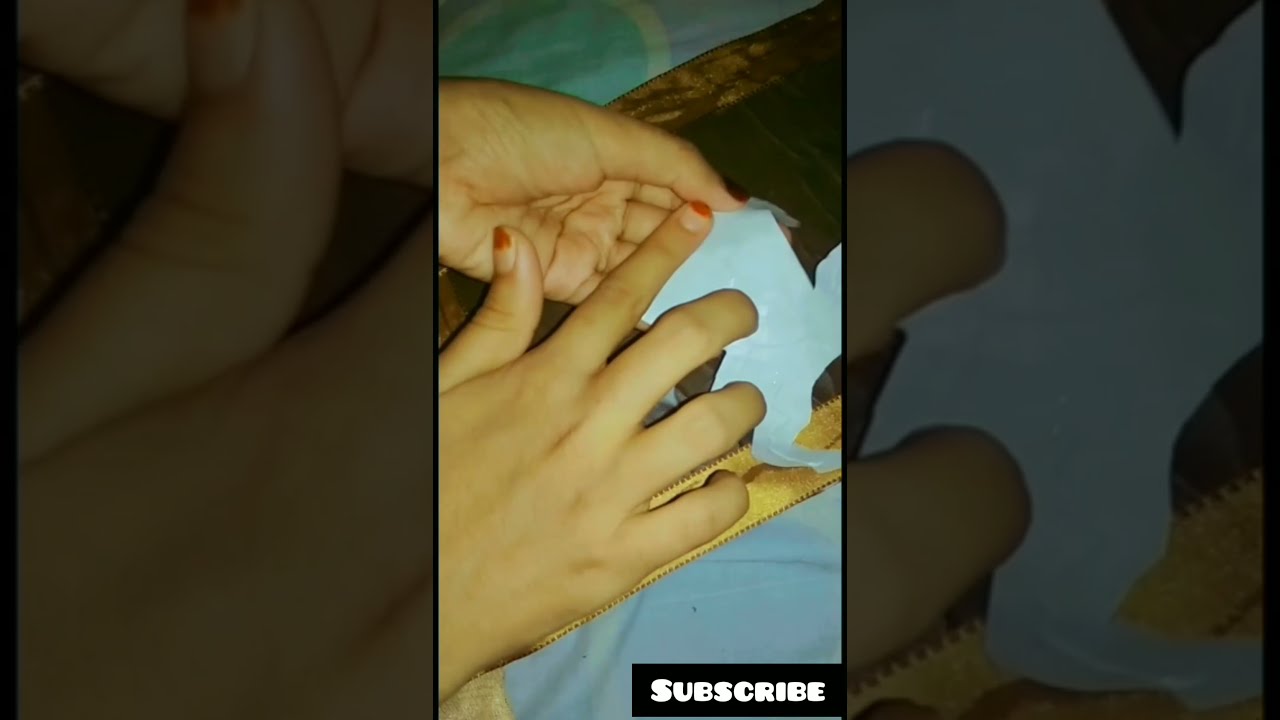This wide rectangular image features a central tall rectangular photograph of light brown-skinned hands with chipped red nail polish on the thumb and index finger of the right hand. The hands, slightly curved away at the knuckles, are situated against a blue sheet of craft paper. The right hand appears to be working with fabric, while the left hand, positioned towards the top left, cups the blue paper. Next to the central image, on both the left and right sides, are darker, wider rectangles containing close-up, shaded images of the central photograph, adding contrast and depth to the composition. At the top of the image, a green object is partially visible. In the bottom right corner, a black rectangle reads "subscribe" in white font, suggesting this might be a screenshot or advertisement for a channel. The overall color tone of the image is fairly yellowish, with details like gold trim on the fabric and faint dotted lines hinting at digital editing.